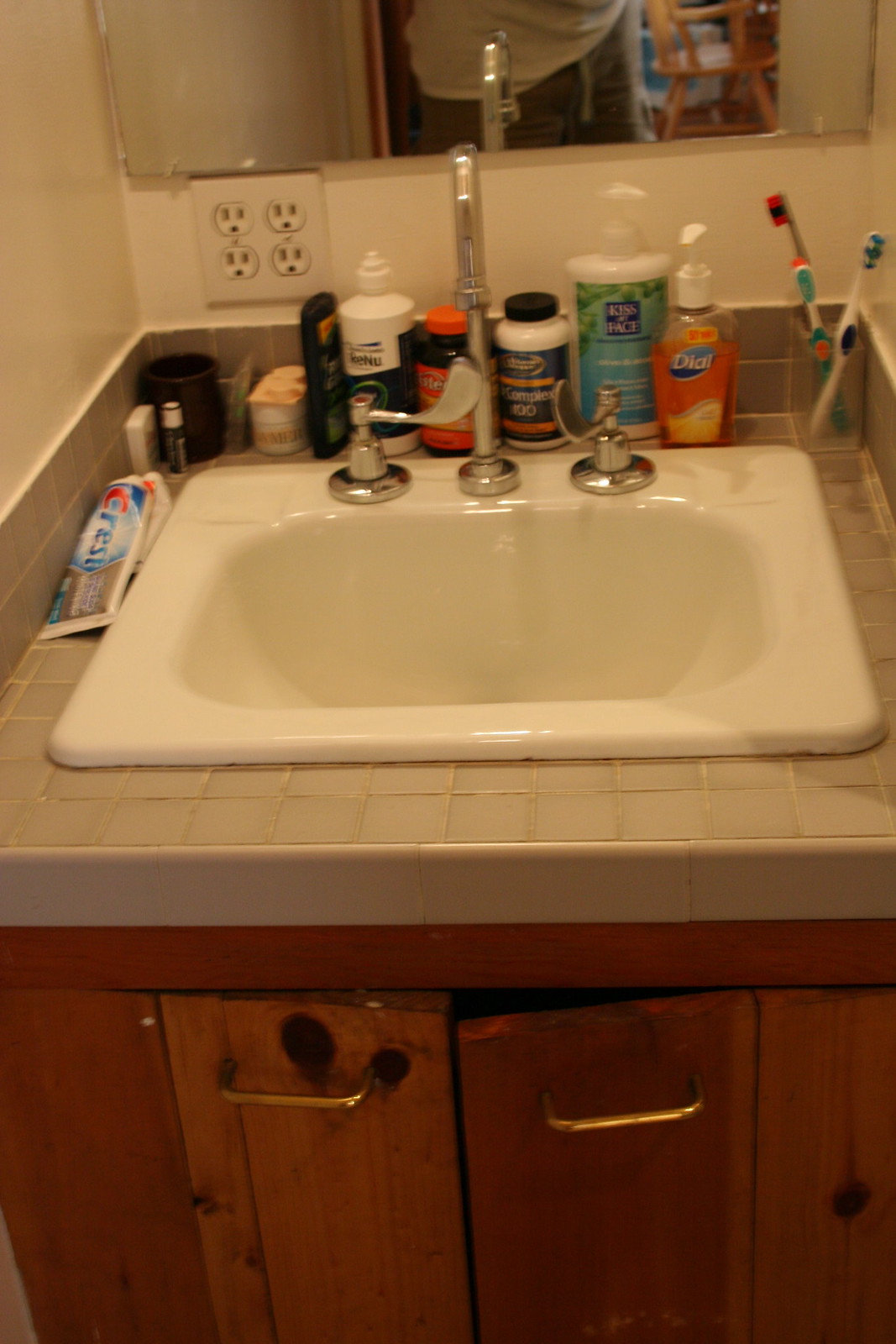A detailed photograph showcases a traditional, old-style bathroom sink with a deep, ceramic basin. Below the sink, there is a wooden cabinet with horizontal gold-plated handles. The handles appear to be metal and securely nailed in place. The base surrounding the sink is adorned with tiles, adding to the vintage aesthetic. On the right side of the sink, two toothbrushes, toothpaste, lip balm, and a bar of soap are neatly arranged. An electric outlet is visible on the left side. Above the sink hangs a mirror that reflects the person taking the photograph. The sink is equipped with silver faucets, completing the timeless look of the bathroom setup.